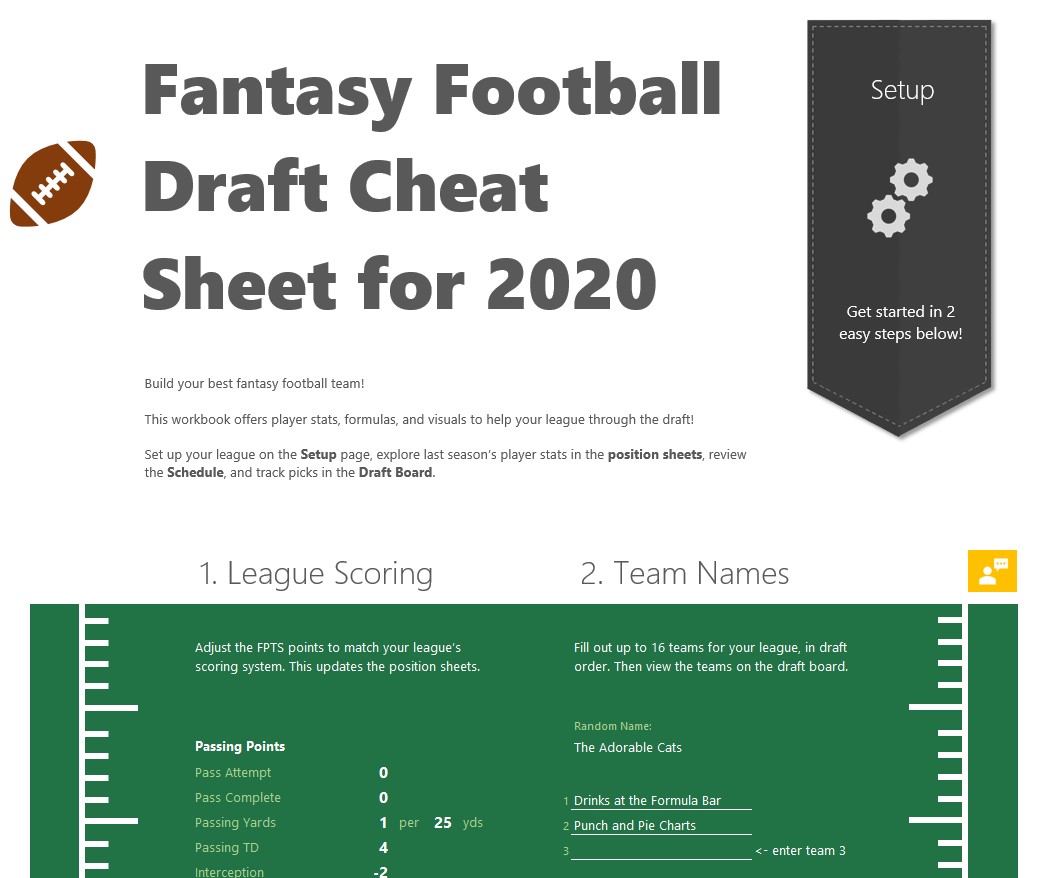This image serves as a detailed fantasy football draft cheat sheet for 2020, predominantly set against a green background with a plethora of white text. Dominating the top center in large dark gray font is the title, "Fantasy Football Draft Cheat Sheet for 2020", accompanied by a small brown football icon to the left. Below this, in slightly smaller text, are the instructions "Set up getting started in two easy steps". The first step is "League Scoring", and the second is "Team Names".

Additionally, there is a vertical banner on the right side featuring white text that begins with "Set up", accompanied by an icon of two cogs. This section provides a concise guide: "Build your best fantasy football team. This workbook offers player stats, formulas, and visuals to help your league through the draft". Detailed instructions follow on how to set up the league, explore player stats from the previous season, review the schedule, and track picks. Beneath the main headers, the cheat sheet details "Number one, league scoring" and "Number two, team names", accompanied by a green bar with football field markings, presenting white text for clarity. On the left, it instructs users to "Adjust the FPTS points to match your league scoring system. This updates the position sheets" followed by a list of passing points.

On the right side, it states to "Fill out to 16 teams for your league in draft order, then view the teams on the draft board." Examples of team names such as "The Adorable Cats" are shown, and numbered fields are included, with placeholders like "Drinks at the formula bar" and "Punch and pie charts". The entire layout is digitally created and likely intended for use on a website or advertisement, containing various colors including green, white, gray, brown, black, and touches of orange, making it visually engaging.